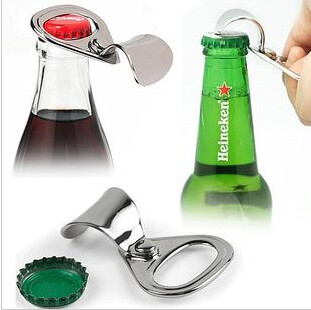This image features a unique bottle opener and its functionality demonstrated on both a Heineken beer bottle and a Coca-Cola bottle. The bottle opener is designed to resemble a pop top from a can, complete with a curved end and an opening loop that mimics the tab you'd pull on a can. In the foreground, the sleek and modern-looking opener, made from a seemingly durable metal, is shown in its entirety. The opener's versatility is showcased through its ability to open bottles using either end: the loop part for a Coke bottle and the curved part for a Heineken bottle. Adjacent to the opener, there's a green bottle cap, emphasizing its practical use. The image also includes the neck and top portion of both the Coca-Cola bottle and the Heineken bottle, illustrating how the opener functions with different types of bottles. The Heineken bottle is particularly noted for its contemporary, shiny appearance with distinctive ridges.